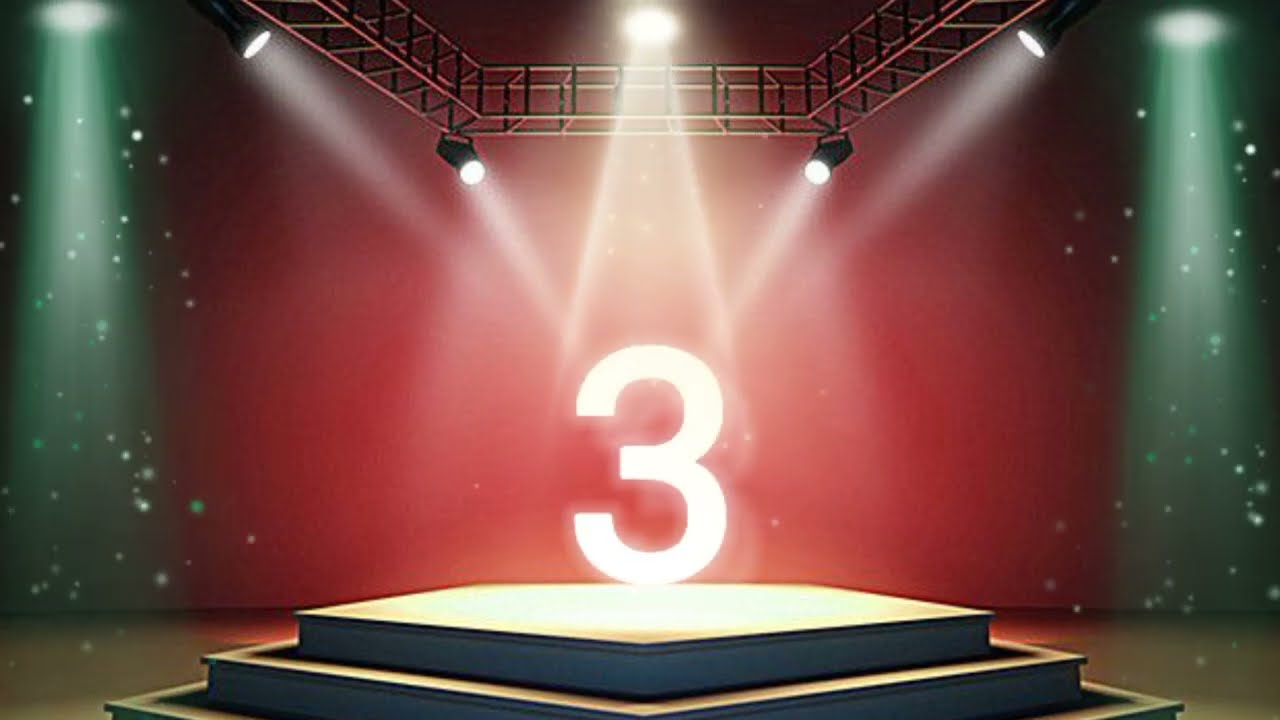This digital artwork features a vivid, computer-generated stage scene with a bright red background that transitions to black near the edges. Flanking both sides of the scene are two luminous green orbs that cast light downward. The floor is light brown, and set prominently in the image's center is a pedestal with three tiers, shaped in a polygonal, four- or five-sided design for each step. On top of this pedestal, a neon-bright, white number three stands out strikingly. Overhead, a piece of scaffolding supports five black spotlights that shine directly down onto the number three, highlighting it with white light. Additionally, in the upper left and right corners, two more green spotlights cast their beams downwards. The background is adorned with sparkling stars and fairy dust, adding a magical atmosphere to the scene. The viewpoint is level with the stage, offering a straight-on perspective of the intricate setup.